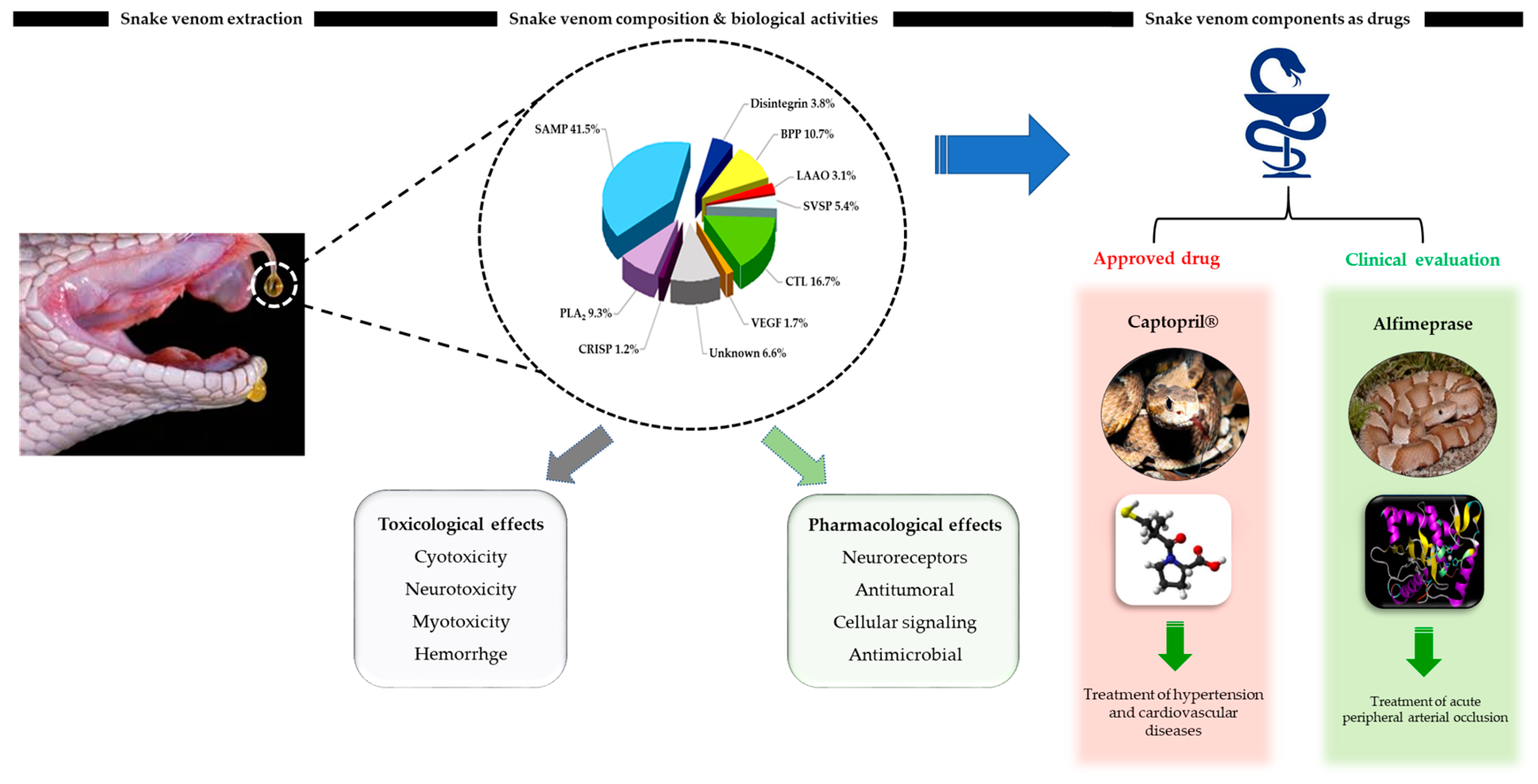This informational image presents a scientific analysis of snake venom through detailed visual elements and text. At the top, it introduces three main sections: "Snake Venom Extraction," "Snake Venom Composition and Biological Activities," and "Snake Venom Components as Drugs," each separated by black bars. The first section features a close-up photograph of a viper's open mouth with venom visibly dripping from its fangs. This transitions into a pie chart illustrating the various components of the venom. 

The next section breaks down the toxicological and pharmacological effects of these components, listing terms such as cytotoxicity, neurotoxicity, myotoxicity, hemorrhage, neuroreceptors, antitumoral properties, cellular signaling, and antimicrobial effects. In the final section, a symbolic image of a snake coiling around a medical rod is shown, which separates the approved drugs from those under clinical evaluation. The approved drug, highlighted in a pink box, is Captopril for treating hypertension and cardiovascular diseases. Meanwhile, Alfimeprase, intended for the treatment of acute peripheral arterial occlusion, is shown in a green box under clinical evaluation. This comprehensive layout effectively communicates the multifaceted research and therapeutic applications of snake venom.